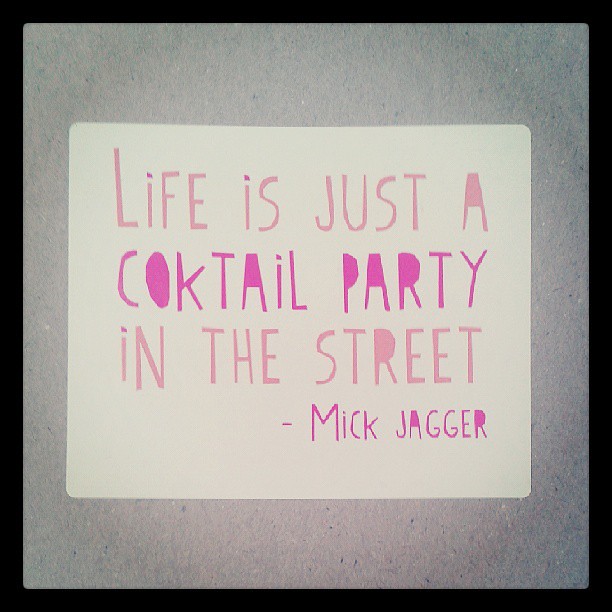The image features a rectangular piece of white paper with a grainy texture and a surrounding thin black border. This white paper is overlaid on a gray, slightly dirty-looking background that includes hints of green, blue, and black. The paper contains an inspirational quote written in markers, with varying shades of pink. The text is somewhat unevenly sized, as though hand-drawn, with some letters colored in or capitalized inconsistently.

The quote reads, "Life is just A COKTAIL party in the street," followed by "Mick Jagger" at the bottom. The word "cocktail" is misspelled as "COKTAIL." All letters are predominantly in uppercase except for the dotted 'i's, which are in lowercase. Specific letters like 'O,' 'A,' 'P,' and 'R' in the quote are filled in with darker pink, emphasizing their shapes. The quote is spread over four lines:

1. "Life is just A" in light pink, with the last 'A' partially colored in.
2. "COKTAIL party" in darker pink, with the 'O' completely colored in and the 'I' lowercase.
3. "in the street" mainly in light pink, except for the lowercase 'i' and the 'R' colored in dark pink.
4. "Mick Jagger" written in darker pink, the 'A' and 'R' partially colored in, and the 'i' lowercase.

The overall aesthetic of the image suggests a handmade, artistic vibe, with emphasis on the playful and imperfect nature of the text's presentation.